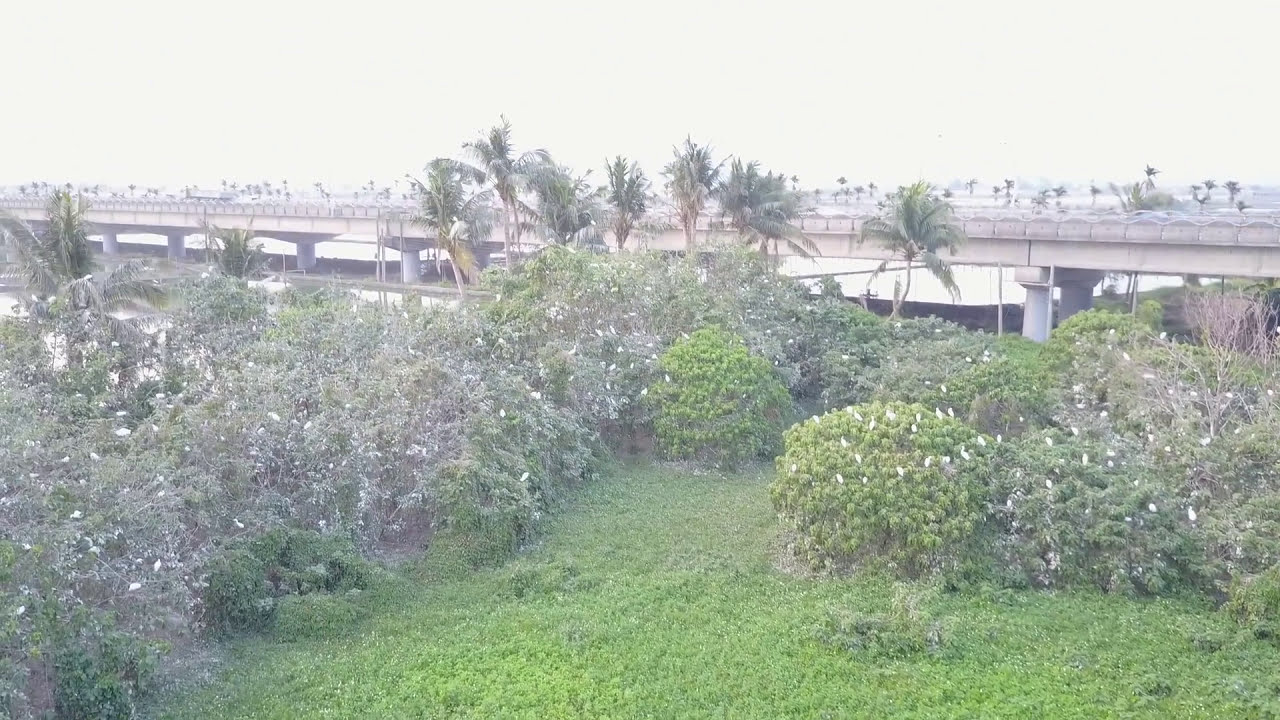The image captures a washed-out, overexposed scene featuring an overpass bridge supported by heavy pylons, stretching from left to right. In the foreground, a variety of vegetation is present, including several sparse bushes adorned with white flowers, along with patches of green ground cover. Taller palm trees are interspersed among the bushes, standing closer to the overpass. The bridge itself is likely a roadway for vehicles, though it has the appearance of a train track due to its pylon supports. The sky above is difficult to discern due to the overexposure, but it suggests either a clear or overcast day. The middle ground features a flat area with grass surrounded by the aforementioned bushes. Palm trees also appear in the distant background, lining the far edge beyond the bridge. The overall color and detail are muted and challenging to distinguish due to the image's high exposure level.